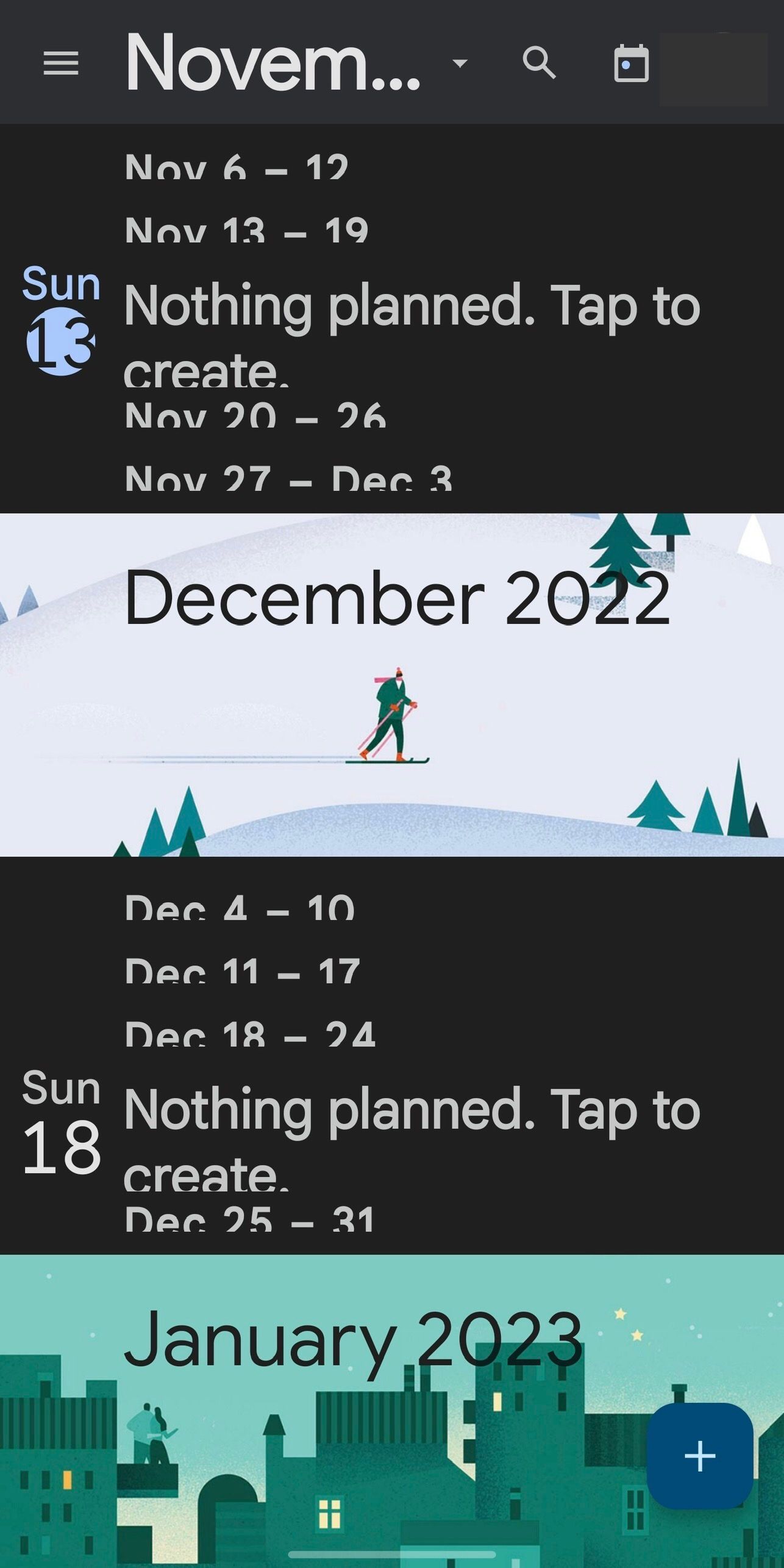A cell phone screenshot features a predominantly black background. In the upper left corner, there are three white horizontal lines indicating a menu icon. To its right, the word "NOVEM" is displayed in large white letters, followed by three dots. Adjacent to this, a small white magnifying glass icon and a calendar icon are visible.

Below these icons, a black rectangle occupies the screen, displaying the word "Sun" in blue on the left side. Beneath "Sun," a blue circle contains the number "13" in black. To the right of this, in large white letters, the text "Nothing planned. Tap to create." is prominently featured. This message is flanked above and below by partially visible dates, such as "November 6-12" and "November 13-19," appearing on a scrollable wheel interface.

Further down, there is a light gray rectangular section. Centered at the top of this section, "December 2022" is written in black. An image of a skier, flanked by green pine trees and snow-covered hills, is displayed below the heading.

Following this, another black rectangle shows rolling dates from "December 4-10" to "December 25-31." Centered on the left in white text, it reads "Sunday," followed by the number "18." Slightly below, the phrase "Nothing planned. Tap to create." is visible once more.

At the bottom of the screenshot, a final rectangle features the text "January 2023" at the top, set against a light sea green background. Below this are green buildings completing the scene.